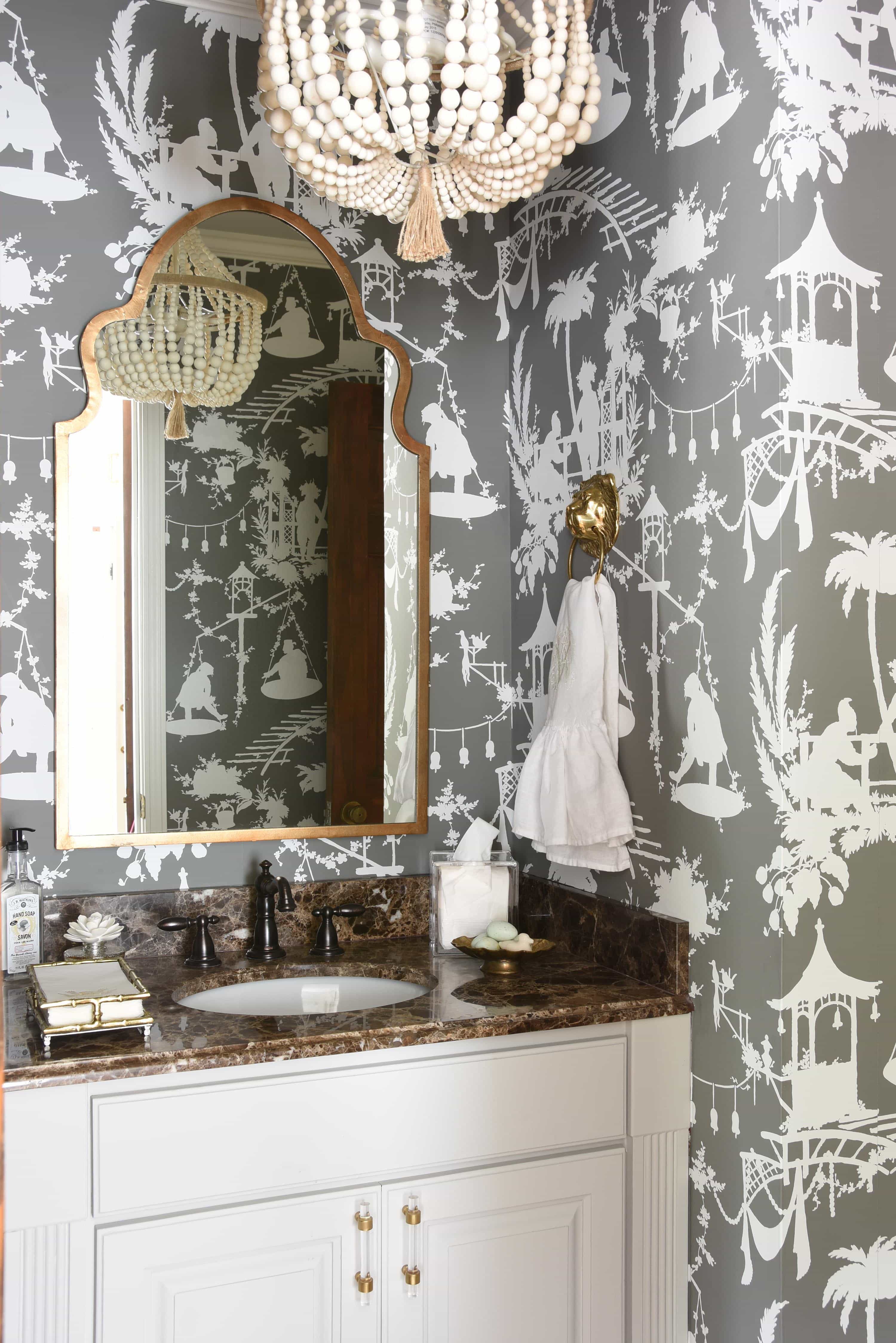This is a photograph of an ornate powder room featuring an intricate gray wallpaper adorned with white images depicting bridges, houses, geishas, and people in various activities such as drinking tea in a garden. The wallpaper sets a sophisticated tone with its rich, Oriental-inspired design. Below the wallpaper, a luxurious granite countertop in hues of brown and black houses a modern black faucet with matching handles. The sink area is equipped with a soap dish, fancy paper towels, a lucite tissue holder, and a glass bottle, possibly lotion, arranged neatly on the countertop. A gold-trimmed mirror hangs above the sink, reflecting the elegant surroundings. To the side, a golden lion-faced ring holds a pristine white towel. The white cabinetry under the sink features two pull-out doors, contributing to the room's polished look. Overhead, a beaded chandelier light fixture adds a final touch of elegance to this meticulously decorated space.